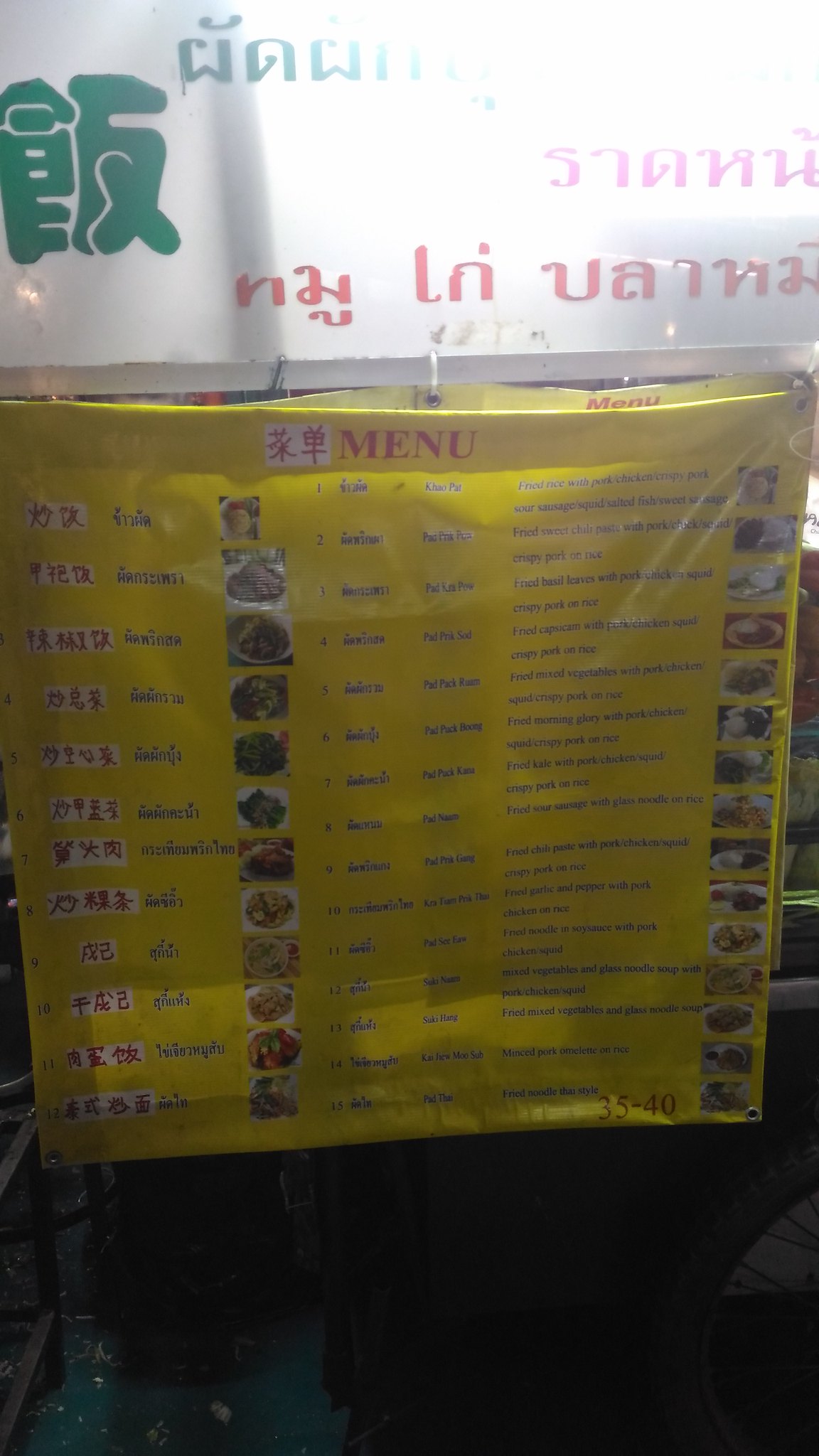This image captures a slightly blurry menu posted inside an Oriental food restaurant. The menu is prominently displayed beneath a frosted glass window, positioned in such a way that its bright yellow background and title—'Menu'—stand out. The window above features intricate red Oriental letters written in reverse, adding a touch of authenticity and cultural flair. In the upper left corner of the window, there is a green emblem or symbol that further accentuates the restaurant's traditional aesthetic.

The menu itself is organized into two columns, each consisting of multiple menu items, although the text is illegible due to the blurriness of the image. Each menu item is accompanied by a small square photograph, providing a visual representation of the dish, followed by the price. The menu is securely fastened to the window using metal clips, making it easy for patrons to peruse from both inside and outside the restaurant.